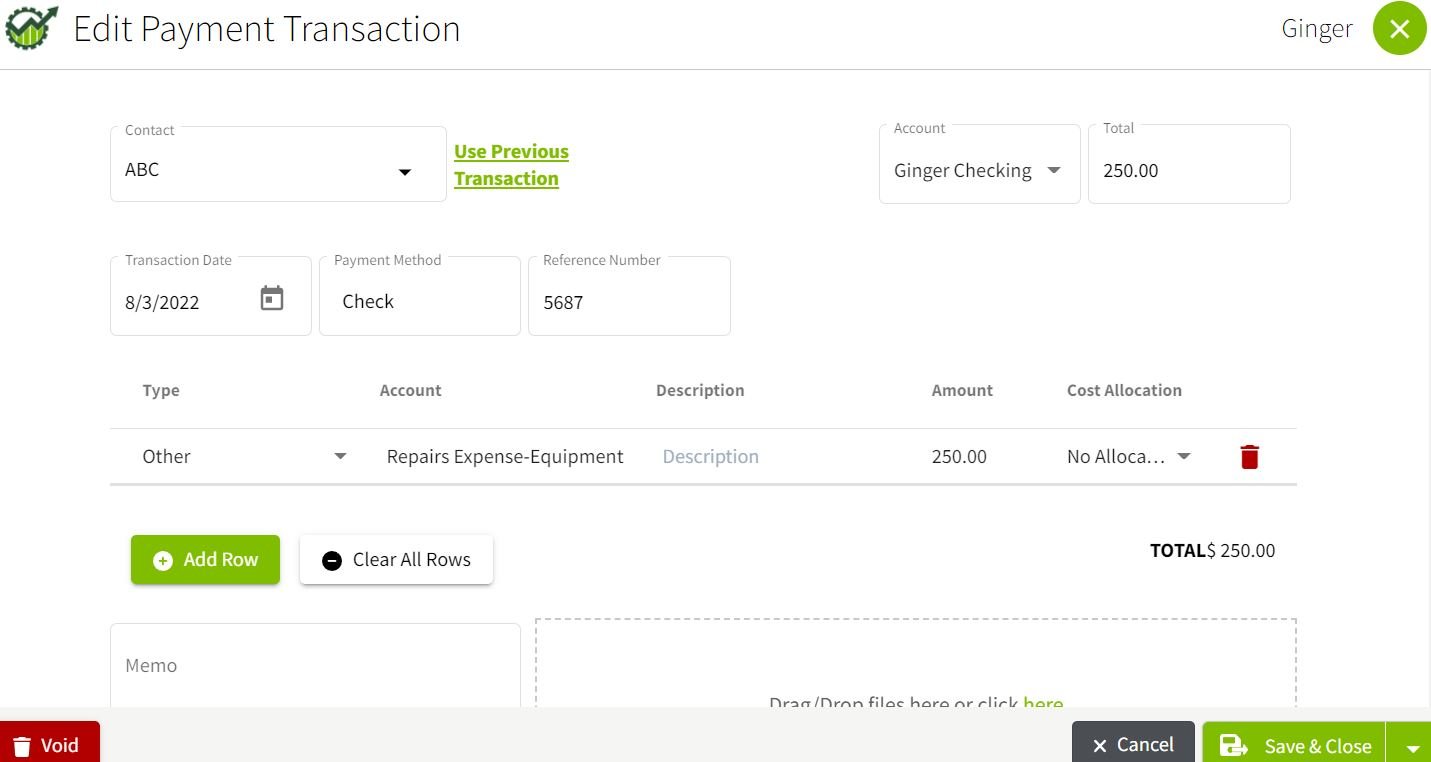Screenshot of a Payment Transaction Editor Interface

This image captures a screenshot from a payment transaction editor interface. At the top of the interface, the title "Edit Payment Transaction" is prominently displayed. On the top right corner of the screen, there is an "X" button, labeled "Ginger," which suggests a user or session identifier.

The main content area lists the details of a specific transaction. Key fields include:

- **Contact:** ABC
- **Account:** Ginger Checking (with an adjustable option to select a different account)
- **Total Amount:** $250.00
- **Transaction Date:** August 3, 2022
- **Payment Method:** Check
- **Reference Number:** 5687

Further below, the interface is organized into a column table with headers such as Type, Account, Description, Amount, and Cost Allocation. The table entries are as follows:

- **Type:** Other
- **Account:** Repairs, Expense, Equipment
- **Description:** None
- **Amount:** $250.00
- **Cost Allocation:** None

Additional action buttons include "Add Row" and "Clear All Rows," placed below the table. On the right side of the interface, the total amount is reiterated as $250.00.

There's also a link labeled "Use Previous Transaction" for potentially reusing transaction details in future entries.